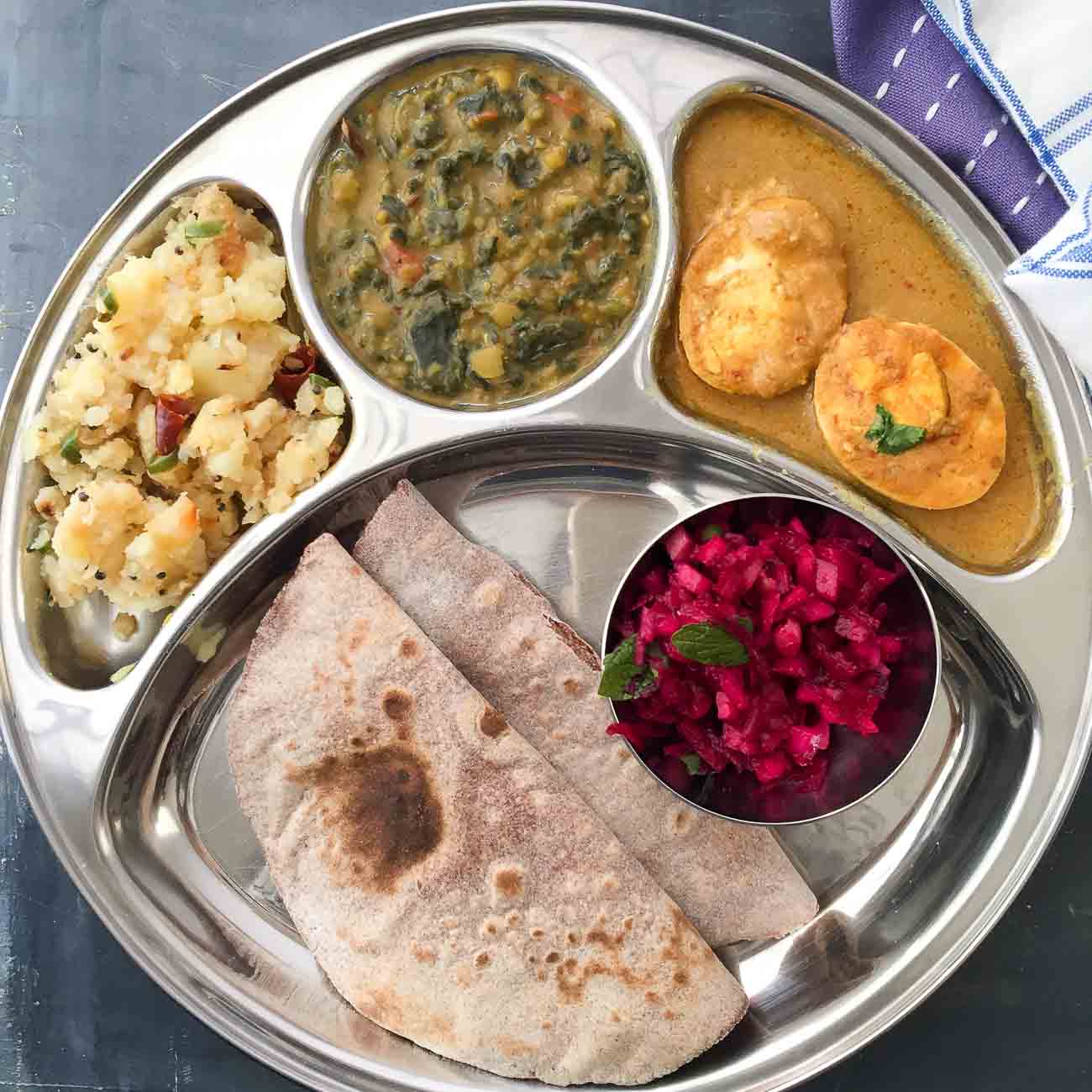This vertical rectangular image features a metal plate with four distinctive compartments, each filled with a variety of food items. The plate is an oval shape that tapers to a point at the bottom. The largest compartment at the bottom holds what appear to be two folded tortillas or tamales. Adjacent to these is a small stainless steel cup containing a red relish or chopped condiment, possibly cranberries or pickled beets. 

In the upper left small compartment, there is a collection of vegetables, likely mashed potatoes or cauliflower bits. The central compartment above contains a salsa-like mixture with a noticeable medley of colors. The upper right compartment showcases what seems to be a sliced hard-boiled egg resting in a distinctive sauce, which could be curry-based.

The entire presentation is vibrant and detailed, indicating a potentially hospital setting, discernible by a glimpse of a blue and white bed sheet in the upper right corner. The food is attractively plated, contradicting initial assumptions of institutional food, and showcases a balanced assortment of textures and flavors.